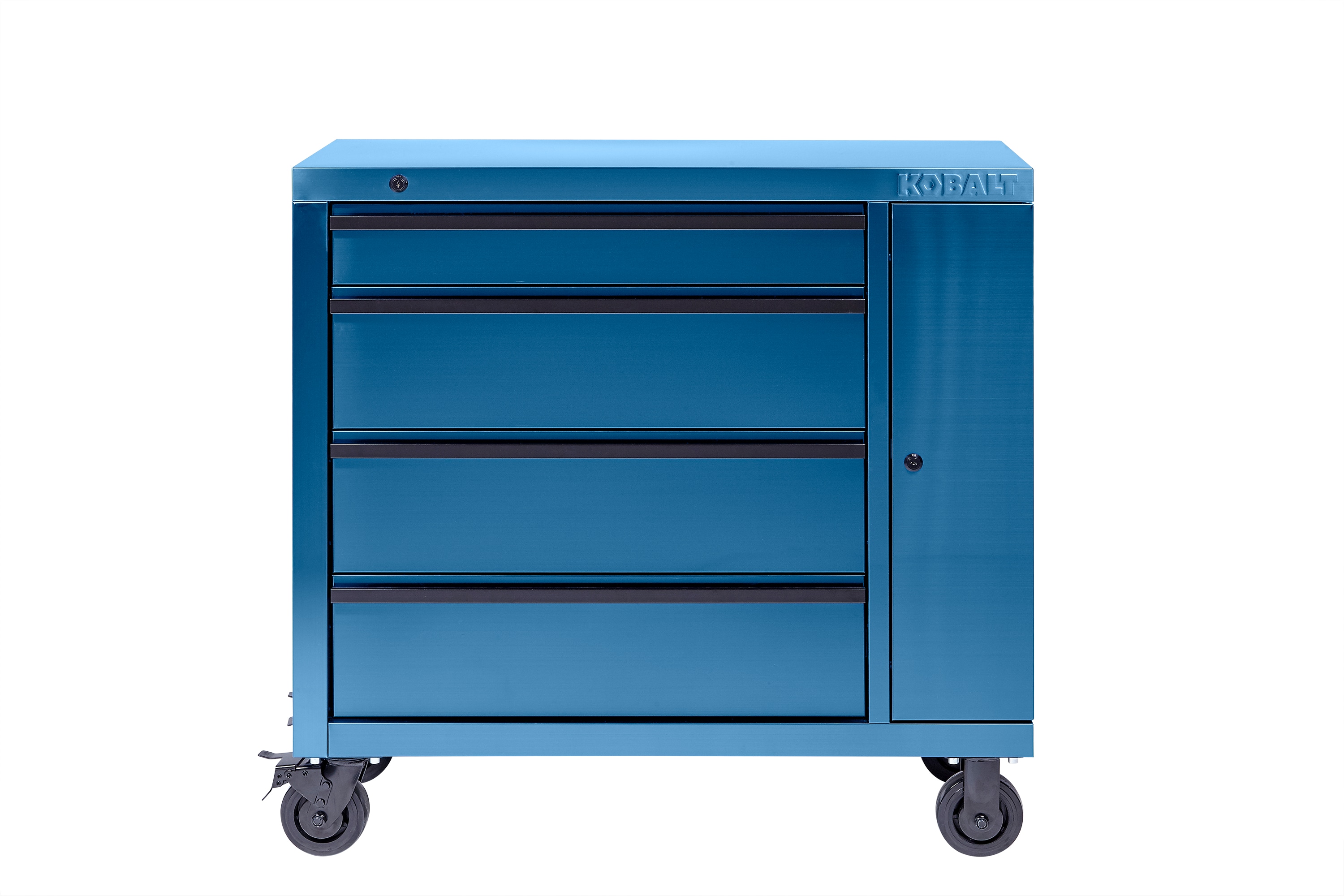This is a detailed front-facing view of a mechanics tool chest by Cobalt, placed against a white background. The tool chest is predominantly a medium blue color, exhibiting a gradient from light blue at the top and bottom to darker blue in the middle. The brand logo "Cobalt" is embossed in a slightly lighter blue on the upper right corner of the chest.

The chest features a total of four rectangular drawers: the top drawer is the thinnest, while the three below it are progressively larger, with the bottom two drawers being nearly identical in size. Each drawer has a black rim serving as the handle. To the right of these drawers is a slender cabinet, running the full height of the chest, and is equipped with a black keyhole in its center.

The tool chest is square-shaped and supported by four wheels at the bottom, which are gray with silver braces connecting them to the structure. The visible part of the wheels is designed for easy rolling, signifying its mobile functionality. This setup suggests a robust and efficient storage solution for mechanics and other professionals, with ample secure storage space in a compact design.